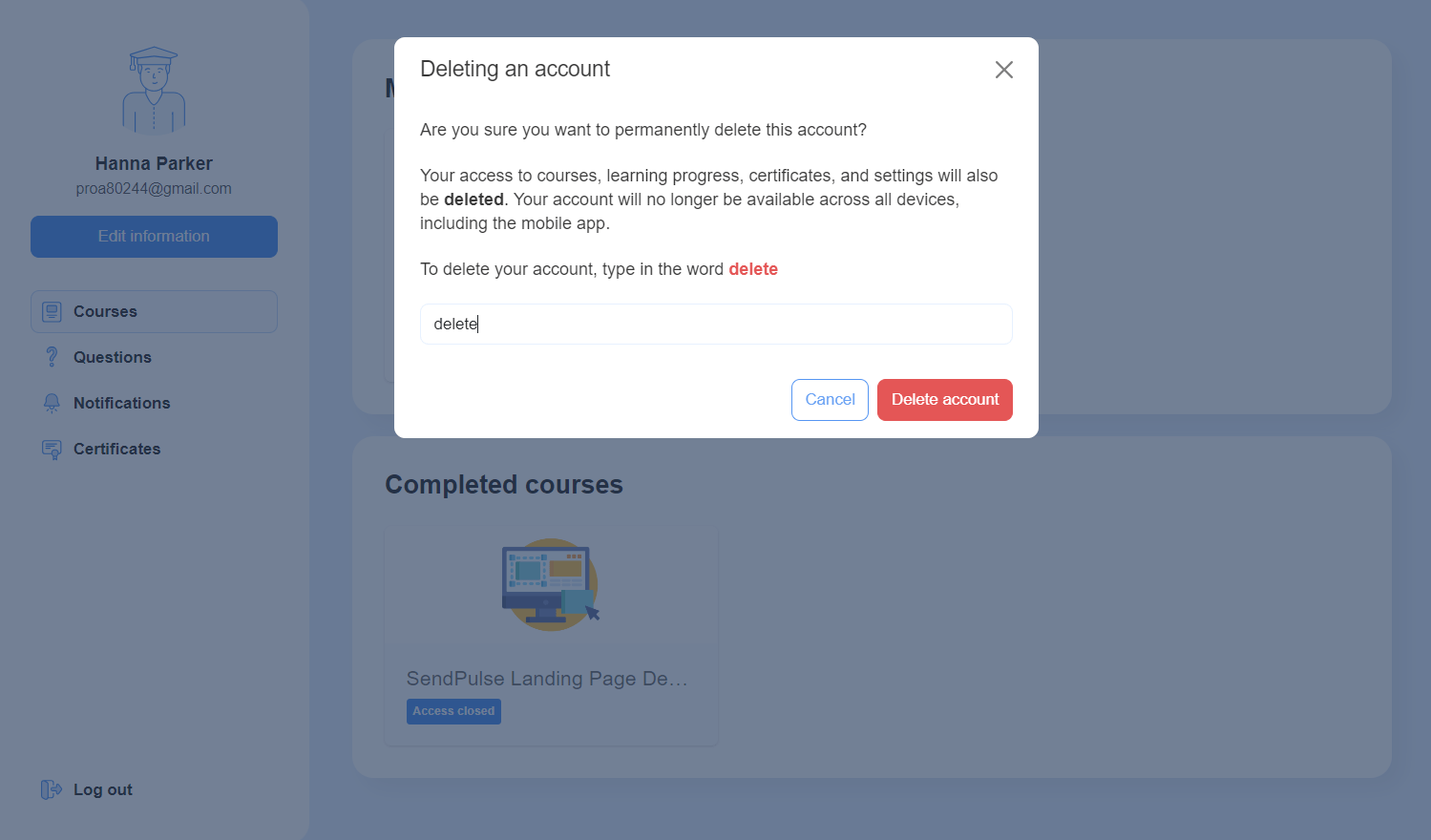In the foreground of the image, prominently displayed, is a large white dialogue box containing a message written primarily in black text. The message reads: "Deleting an account. Are you sure you want to permanently delete this account? Your access to courses, learning progress, certificates, and settings will also be deleted. Your account will no longer be available across all devices, including the mobile app. To delete your account, type in the word DELETE." The word "DELETE" is highlighted in red. Below this instruction, there is a long rectangular input box in which the word "DELETE" has been typed. Beneath the input box, there are two buttons: one is a white button outlined in blue that says "CANCEL," and the other is a red button on the right with the inscription "DELETE ACCOUNT."

In the background, on the left side of the image, there is an avatar depicting the outline of a person wearing a graduation cap. Below the avatar, it reads "HANNAH PARKER PROA80244 at gmail.com." Underneath this, there is a blue horizontal rectangle containing the phrase "edit information." Below, a menu lists "COURSES," "QUESTIONS," "NOTIFICATIONS," and "CERTIFICATES," with "COURSES" highlighted in a muted gray, indicating it is the current selection. The entire background is rendered in a muted gray to draw focus to the white dialogue box in the foreground.

Further in the background, obscured by the white box in the foreground, is another section labeled "COMPLETED COURSES," featuring an icon of a computer monitor accompanied by the text "SEND PULSE LANDING PAGE" followed by "ACCESS CLOSED." In the bottom left corner, the option "LOG OUT" is visible. The context suggests that the user is considering deleting their account, possibly due to graduation or the conclusion of their educational activities within the platform. Some additional elements in the background are partially hidden by the prominent white dialogue box in the foreground.